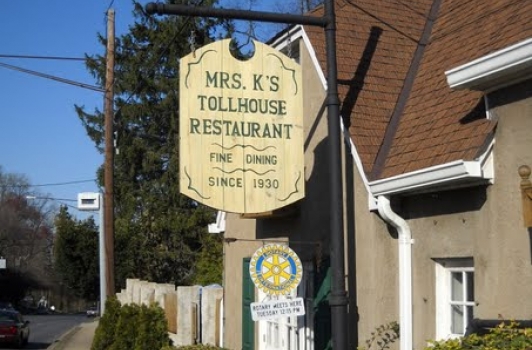This photograph captures an outdoor scene featuring Mrs. K's Toll House Restaurant, a fine dining establishment since 1930. Dominating the center of the image is a yellow wooden sign with green, all-capital letters stating "Mrs. K's Toll House Restaurant", and beneath it in smaller print declaring "Fine Dining since 1930". The sign is suspended from a thin, dark gray metal pole. Below the main sign, there is an additional, somewhat obscured Rotary Club sign featuring a nautical symbol. 

The background showcases a large, well-known pine tree towards the upper left, accompanied by several other green trees extending further up the street, indicating a lush, tree-lined area. The sky is clear and blue, adding to the pleasant ambiance of the setting. To the right of the sign is the restaurant itself, a solid brown stone building with white gutters and window trim, capped with a dark brown tiled roof. Some descriptions mistakenly identify the roof color as red; however, the more repeated observation specifies it as dark brown. Adding to the charm, there's a glimpse of a white picket fence adjacent to the building.

Foreground details include a car driving down the road at the bottom left of the image and a visible telephone pole on a street corner, along with street lighting and posts. The building's old stucco siding, accurately characterized as grayish cream, supports the sign and enhances the overall historical feel of the establishment. Several bushes are present in the scene, contributing to the greenery. There are no people visible in the photograph, focusing the viewer's attention on the architectural and natural elements of the location.